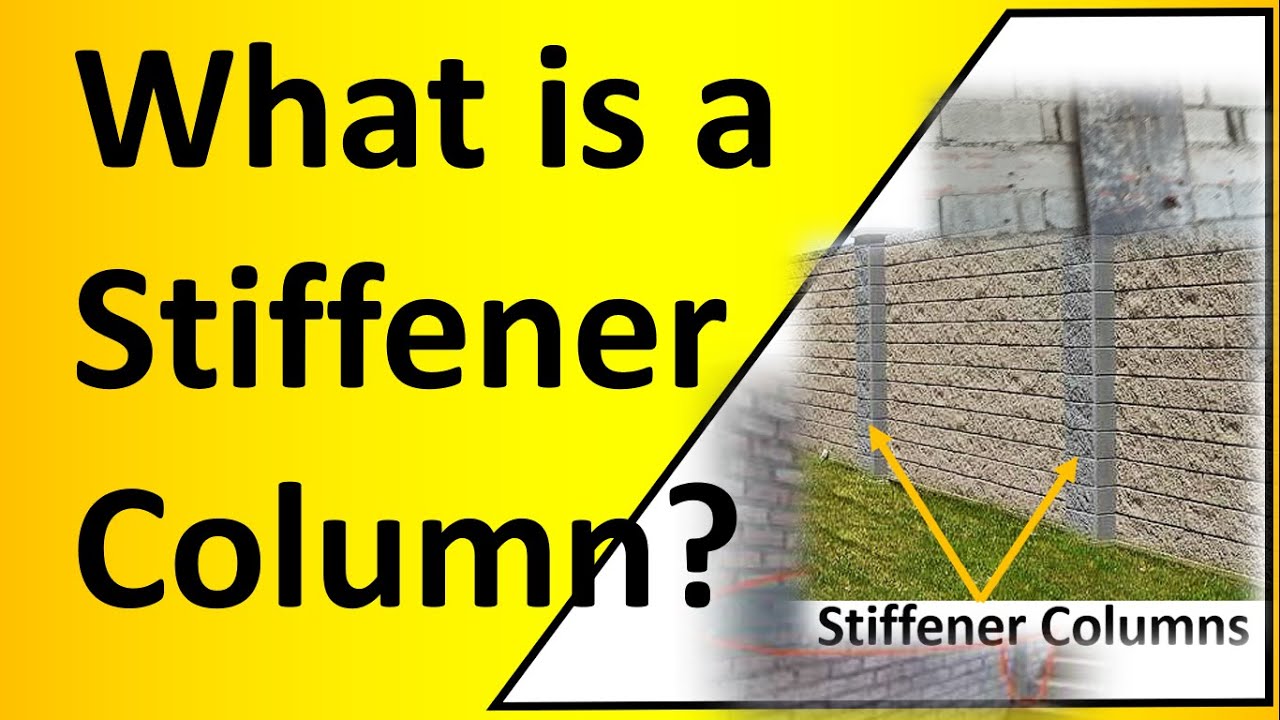The image is an informative ad with a prominent yellow background, oriented horizontally. Across the top, in large black type, the text asks, "What is a stiffener column?" Below this, the words "stiffener column" reappear with an accompanying question mark. To the right side of the ad, there is a trapezoidal cutout featuring a photograph of a stone or concrete wall, which is light brown or cream-colored with horizontally arranged stones. Within this wall, there are two gray vertical columns, labeled "stiffener columns," highlighted by yellow arrows pointing to them from the bottom of the image. These columns, differing in texture and color from the surrounding wall, are depicted to emphasize their structural support function in the building.